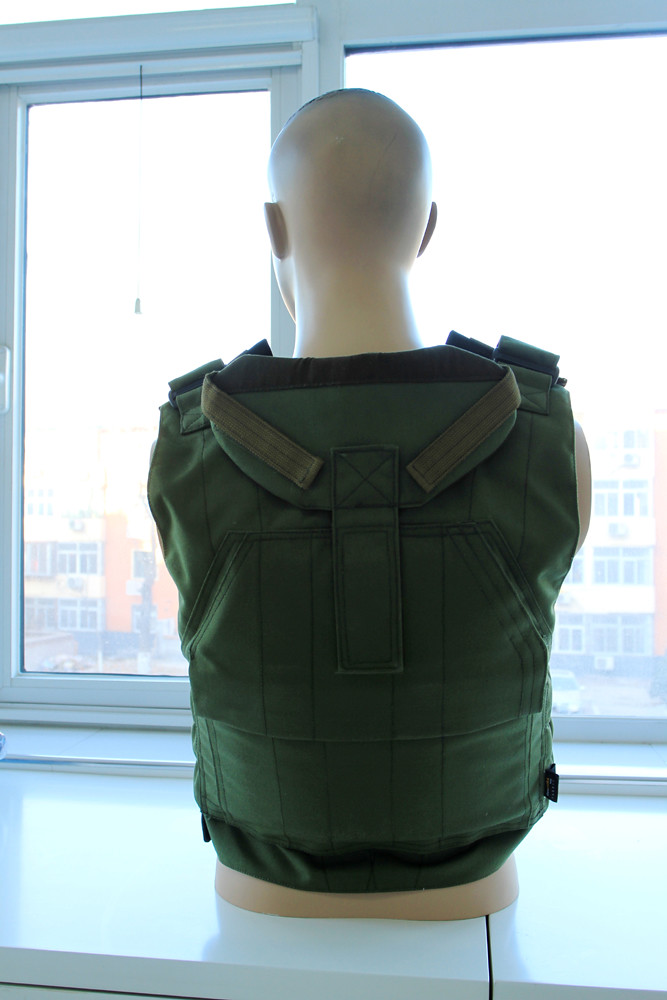This photo captures an intriguing and slightly surreal scene of a male mannequin positioned on a wide marble windowsill, gazing out of a window. The mannequin is only depicted from the waist up, with its lower half absent, creating an illusion that it's more than just a figure. The mannequin wears a military-style, army-green bulletproof vest adorned with various pockets and features, enhancing its lifelike appearance. Its bald head and bare arms are visible, with the back of its ears and neck clearly seen. Through the window, several fog-shrouded, multi-story apartment buildings can be discerned across the street. The window is sectioned with metal frames, adding to the structured aesthetic of the photograph.